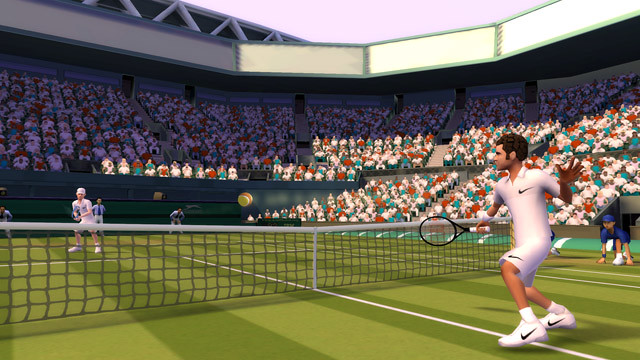This image, likely a screenshot of a high-quality, somewhat realistic video game, captures an intense tennis match set in a stadium reminiscent of a baseball arena. The stadium is filled with spectators clad in turquoise, white, and brick-red attire, seated high in the bleachers under dark green and light green awnings. The open sky above is a striking contrast to the structured layers below. The tennis court itself is a mix of light and dark green hues, marked with white lines and divided by a black net with white edges. On the right side of the image, a player dressed entirely in white Nike gear, including white shoes and socks, stands poised with a black racket, seemingly ready to return a serve. On the opposite side of the net, another player, also in white, is captured mid-serve. The detailed environment, although not photographically precise, powerfully conveys the energy and realism of a live tennis match.